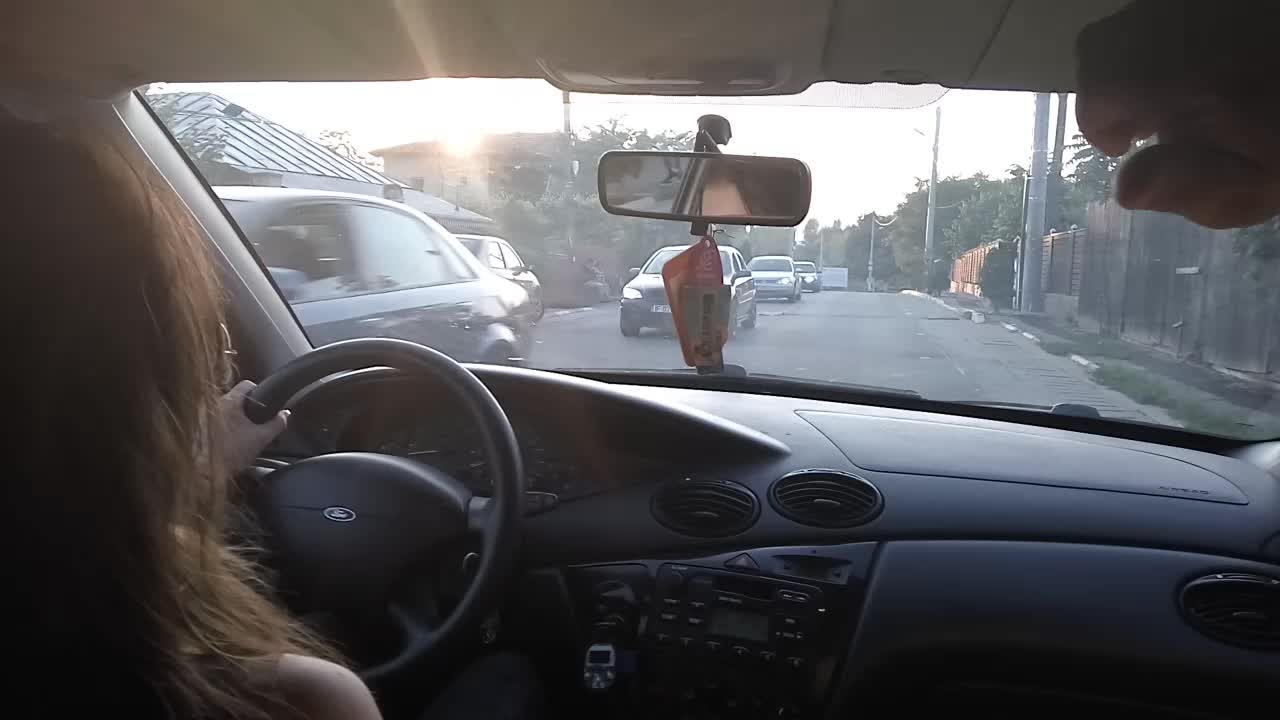A captivating photograph taken from the interior of a Ford car, offers a driver's perspective through the windshield. The driver, a woman wearing glasses, navigates what appears to be an old street with worn sidewalks in a location that might not be the Midwest after all. The scene could potentially be somewhere in another country, perhaps even the Philippines, as suggested by the presence of graceful palm trees swaying gently in the background. The car’s black dashboard and steering wheel frame the view ahead, with oval-shaped bins visible on the dashboard. The golden light of either dawn or dusk floods the image, indicating a serene moment at the beginning or end of the day.